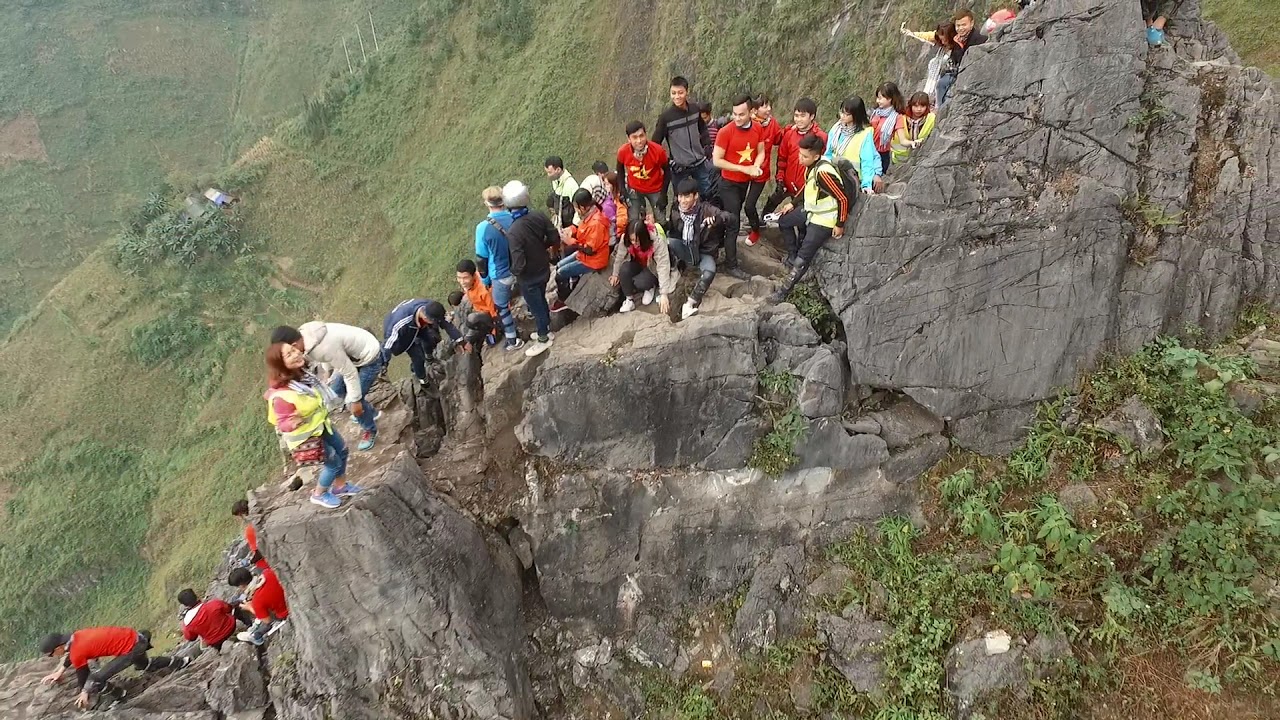A lively group of approximately 30 to 35 people, predominantly Asian, pose together on a large mountainside cliff. The diverse attire ranges from red shirts with yellow stars to blue jackets with yellow scarves, and a standout black sweatshirt with orange stripes on the sleeves. Perched on the flat part of an L-shaped rock, some members of the group lean against the vertical section while others sit or stand. Behind them, grassy, hilly terrain contrasts with the gray stone, painting a vivid scene of their high-altitude rest stop. The steep cliff below reveals a distant structure with a barely visible roof, indicating the towering height of their vantage point. Despite the rugged environment, the group, a mix of young and older individuals, appears relaxed and joyous, laughing and enjoying the bright morning or afternoon sun. They might be on a significant hike, pausing to capture a memorable moment amid their journey.